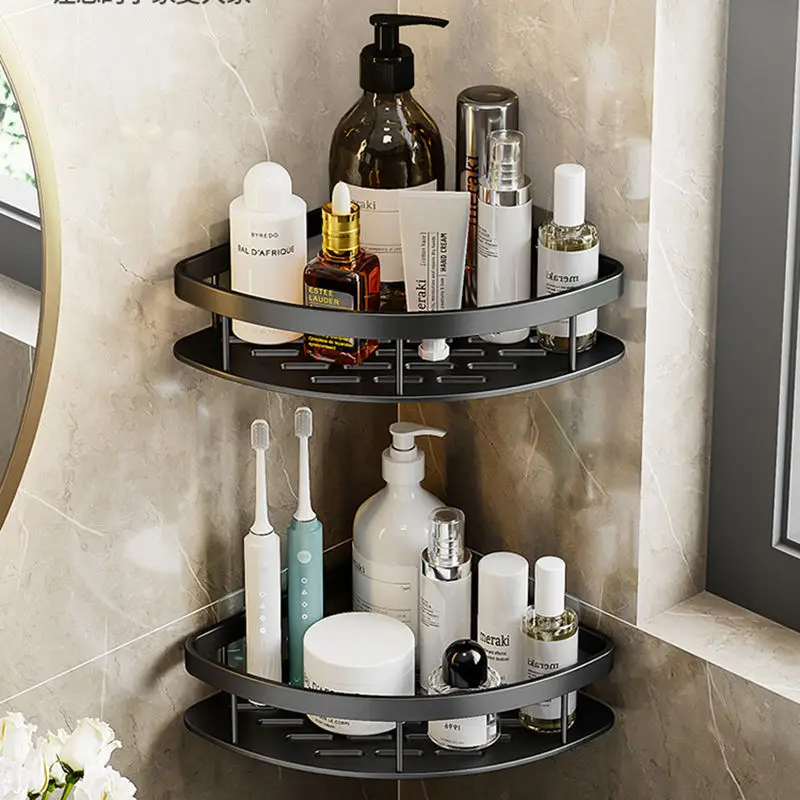In the image, a luxurious bathroom setting is evident, featuring elegant marble walls in light gray hues and a matching marble countertop. Prominently, there is a set of two sleek black metal shelves affixed to the corner of the bathroom wall, likely using high adhesive stickers given the absence of any visible drilling or nails. The shelves have a right-angle design with a curved front, embodying both functionality and style. The upper shelf is adorned with an array of posh, minimalistic makeup and skincare products, exuding a sense of opulence. Below, the lower shelf holds two electric toothbrushes, a bottle of lotion, and various other sundries essential for daily self-care routines. To the left, a glimpse of a gold-rimmed mirror adds a touch of classic elegance, while to the right, a window allows natural light to filter through. A hint of white flowers in the background further enhances the bathroom's serene and sophisticated ambiance.